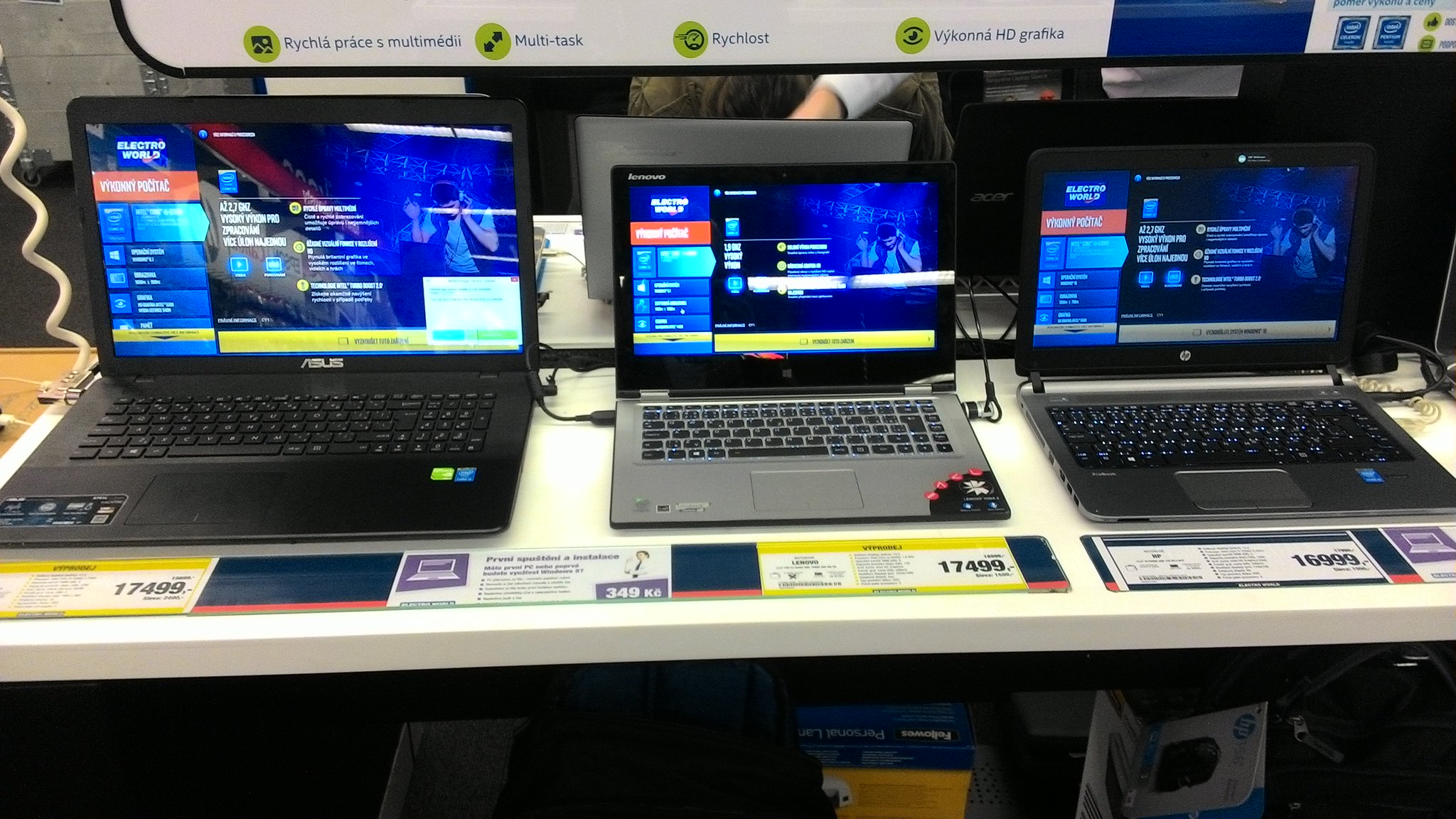This is a vibrant photograph taken inside an electronics store, possibly in a non-English speaking country, showcasing a display of three laptops on a white table. The table features price tags and specification placards in what appears to be Finnish or another Nordic language. From left to right, the laptops are an Asus model in black, a smaller silver-gray laptop, and a medium-sized, darker gray laptop. Each laptop is powered on, displaying a colorful blue splash screen with the word "Electro World" prominently visible. The prices on the tags range from approximately $16,099 to $17,499 in a non-USD currency. The background hints at additional laptops and suggests a bustling store environment, adding to the dynamic, well-lit setting filled with prominent blue hues.